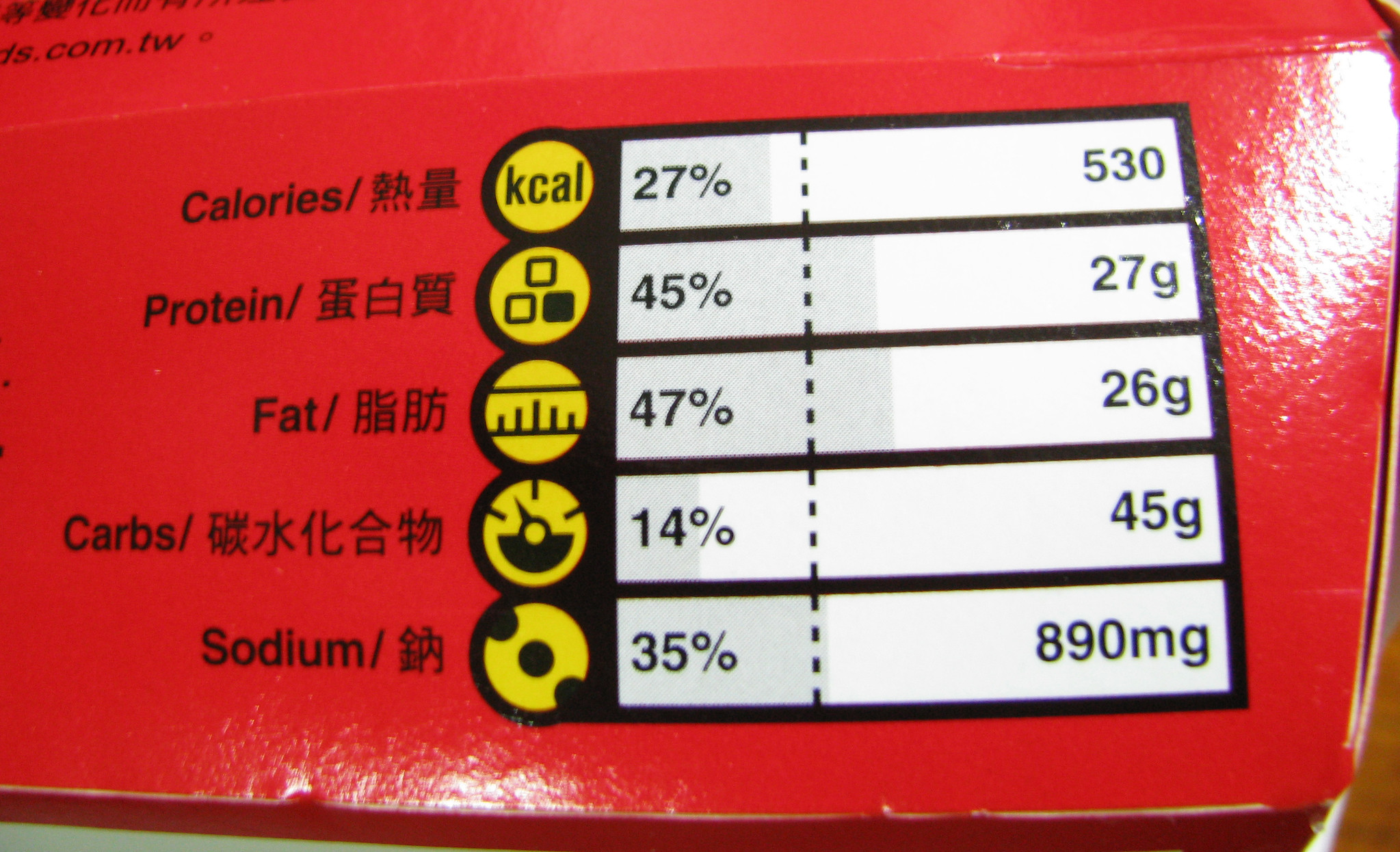This photograph showcases the nutritional information on the back of a high-gloss, red cardboard food or drink container from Taiwan. The package features various components, including calories, protein, fat, carbs, and sodium, each followed by Chinese characters. The calorie content is highlighted as 530 Kcal, representing 27% of the daily value. Protein amounts to 27 grams (45%), fat is at 26 grams (47%), carbohydrates total 45 grams (14%), and sodium is measured at 890 milligrams (35%). The nutritional facts are accompanied by distinct yellow icons, such as a circle for calories, squares for protein, a bar graph for fat, an energy meter for carbs, and three dots for sodium.